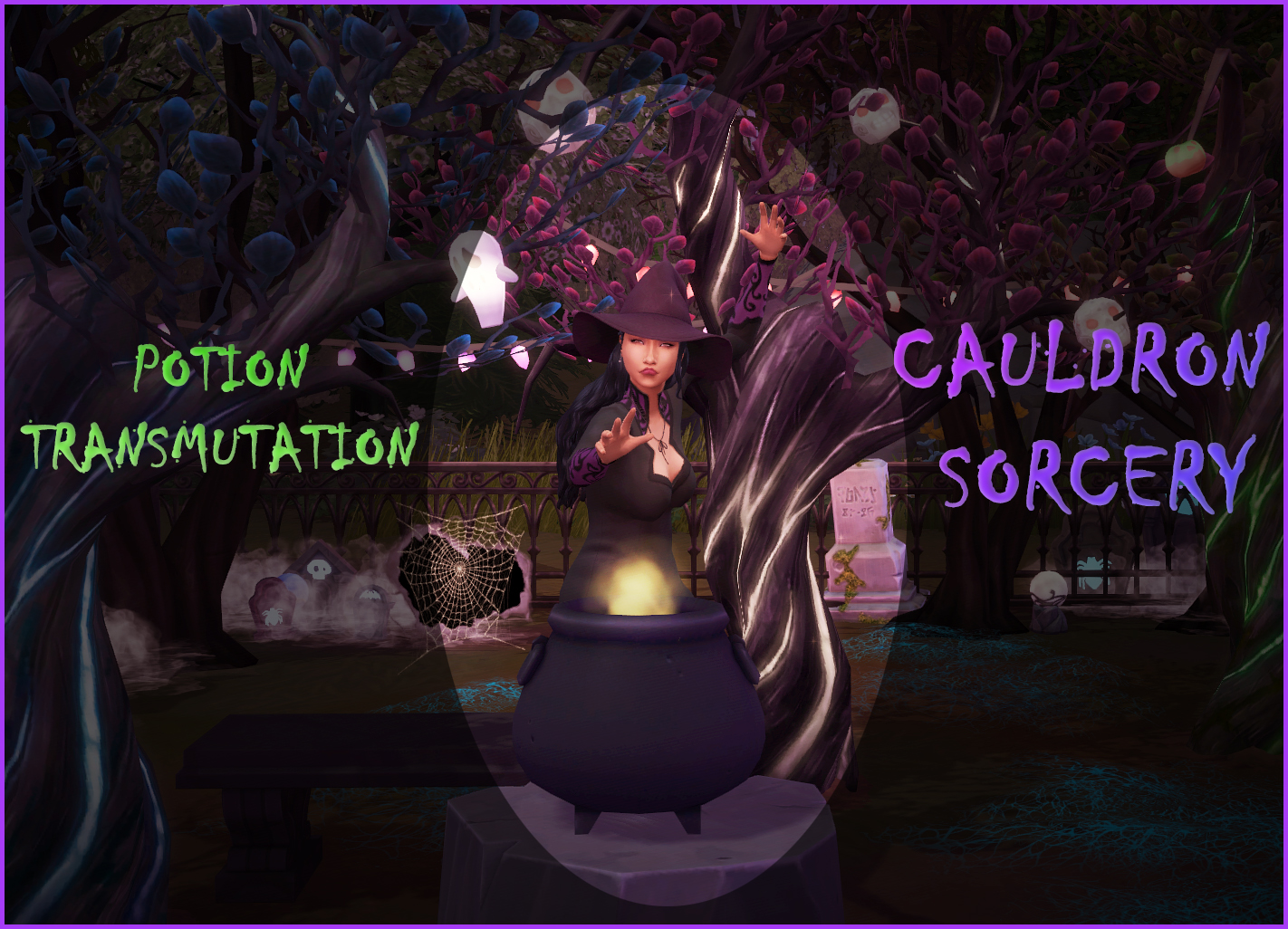This fantasy-inspired, computer-generated poster features a captivating, detailed depiction of a witch in the center, fully illuminated by an oval spotlight while the periphery remains dark and slightly obscured. The witch, donned in a tight, black revealing dress and a pointy hat, stands over a black cauldron set on a stone pedestal, her hands suggestively raised as if casting a spell. The cauldron emits a mysterious, yellowish light, creating an eerie atmosphere. Surrounding the scene are intricate details such as a wooden bench, ornate metal fence, large spiderwebs, and Halloween-themed decorations including gravestones, purple-striped trees, a ghost, and hanging lights. On the left side of the image, green text reads "Potion Transmutation," and on the right, purple lettering spells out "Cauldron Sorcery," each in a unique liquid-splatter-like font that adds a whimsical touch to the dark, magical setting.